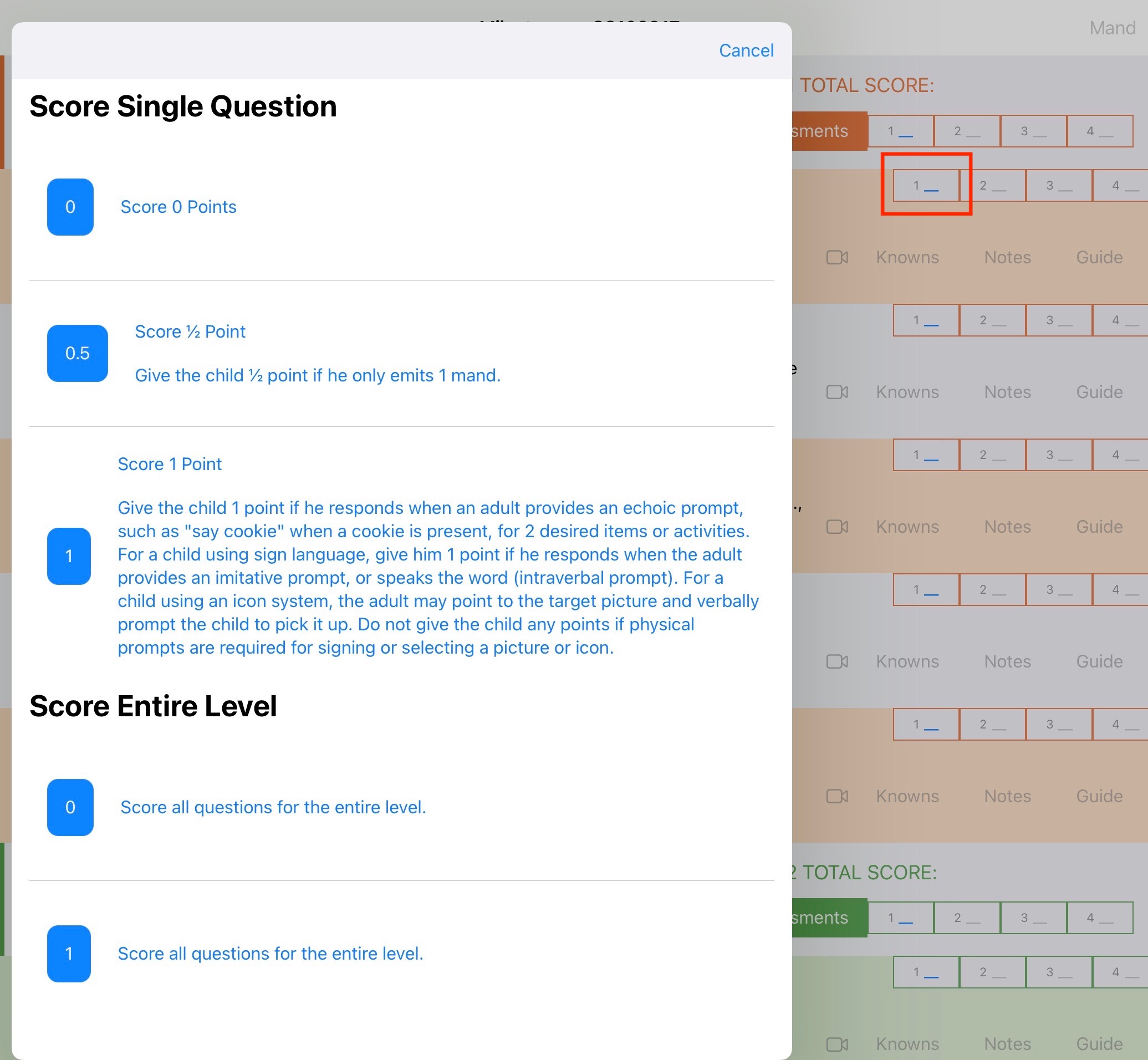The image depicts a website's main page with an overlay pop-up that spans from the left and past the middle to the right side of the screen. At the top of the pop-up, there is a light gray banner featuring the word "Cancel" in blue, capitalized with a capital "C." Below the banner, on a white background, the heading "Score Single Question" is displayed in black text, with "S," "S," and "Q" capitalized.

Beneath the heading, there is a series of blue text enclosed in slightly rounded squares. The first square states "Score: Zero Points." The second square, labeled "Score: Half a Point," contains instructions, giving half a point if the child emits only one "mand" (spelled out M-A-N-D). 

The subsequent square indicates "Score: One Point," providing detailed criteria: one point is given if a child responds to an echoic prompt like "say cookie" when a cookie is present, or responds to two desired items or activities. For children using sign language, one point is awarded if they respond to an imitative prompt. For those using an icon system, the adult may point to the target picture and verbally prompt the child to select it. No points are given if physical prompts are required for signing or picture selection.

Lastly, the pop-up includes a segment labeled "Score Entire Level," instructing to "Score All Questions for the Entire Level." 

This description details the elements and instructions contained within the website's interactive pop-up.